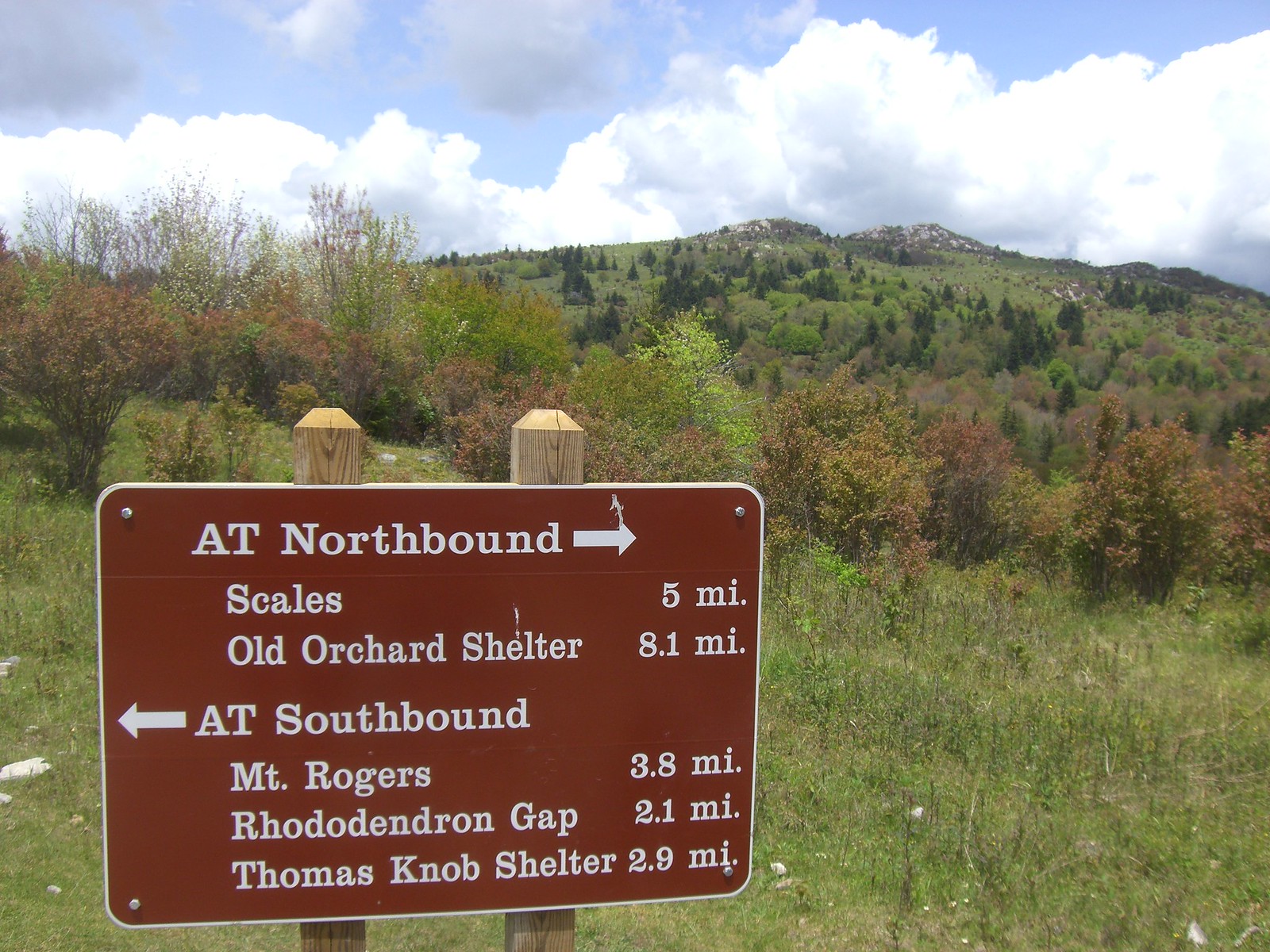This photograph showcases a rustic brown sign mounted on two wooden pillars, prominently featuring white lettering. At the top, the sign indicates "AT Northbound" accompanied by a right-pointing arrow. Below this, it lists "Scales, 5 miles" and "Old Orchard Shelter, 8.1 miles." Further down, "AT Southbound" is marked with a left-pointing arrow, directing to "Mount Rogers, 3.8 miles," "Rhododendron Gap, 2.1 miles," and "Thomas Knob Shelter, 2.9 miles." The sign is situated in a lush grassy field, surrounded by an array of wildflowers, shrubs, bushes, and small trees. In the distant background, rolling green hills and a large grassy slope are dotted with pine trees. The sky above is a vivid blue, populated with white, fluffy cumulus clouds.